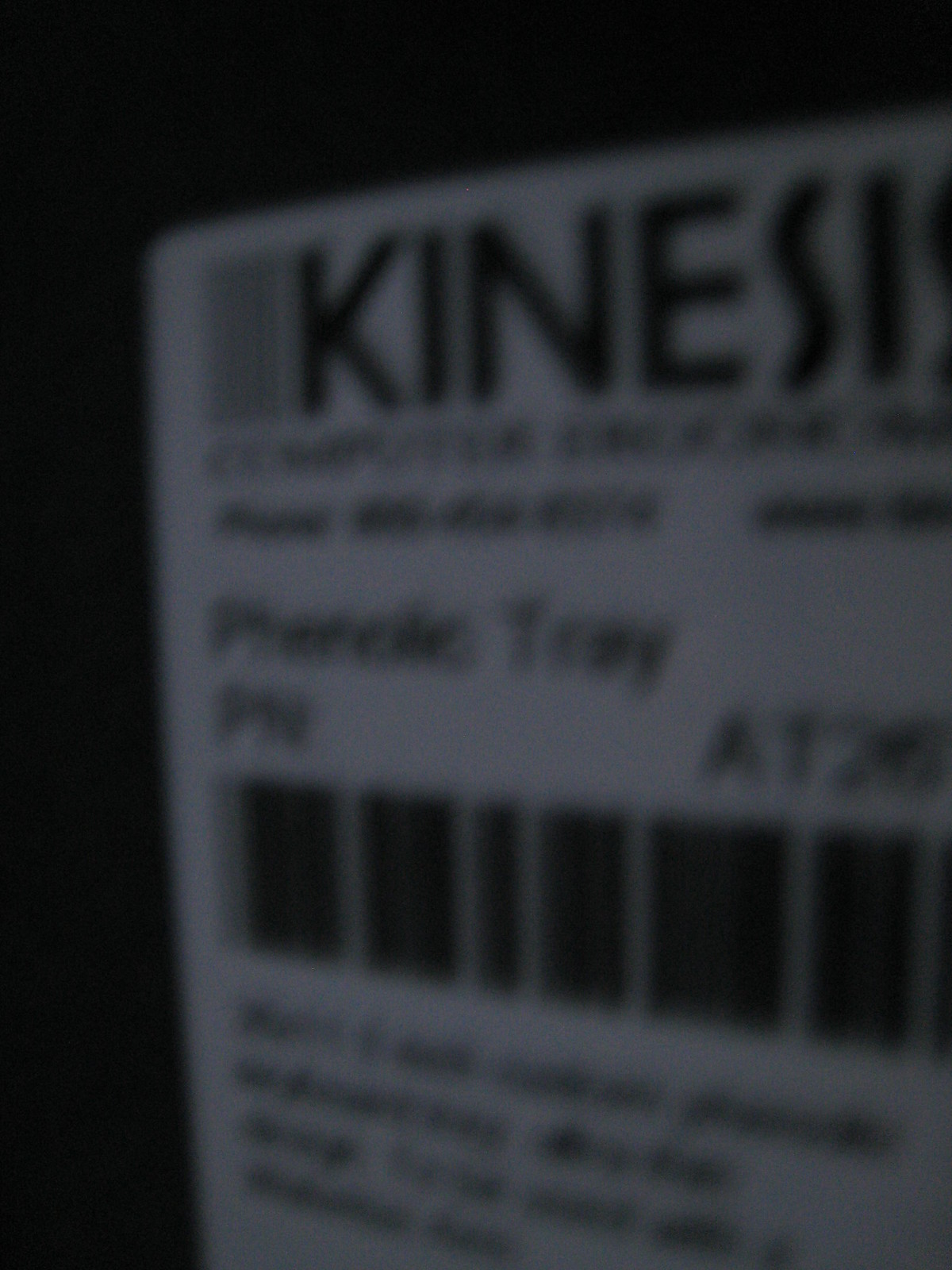The image is a highly detailed, black-and-white close-up of a label or tag set against a very dark background. The label occupies roughly 80% of the photograph, leaving a narrow band of black at the top and left edges. The entire palette comprises shades of black and grey, creating an almost unreal, non-photorealistic texture, either due to an applied dark filter or very low lighting conditions.

At the top of the label, in big capital letters, is the partially legible word "K-I-N-E-S-I." The full word cannot be discerned due to the blurriness of the image. Below this, there's additional text, though most of it is unreadable except for a few decipherable letters: likely forming part of the word "pencilic" or "fensilic," and another word possibly ending in "TRAY". Lower still is a large, vertical barcode, beneath which more text appears, but it remains illegible. The overall contrast between the black and white elements, combined with the inherent blurriness, gives the image a striking yet enigmatic appearance.